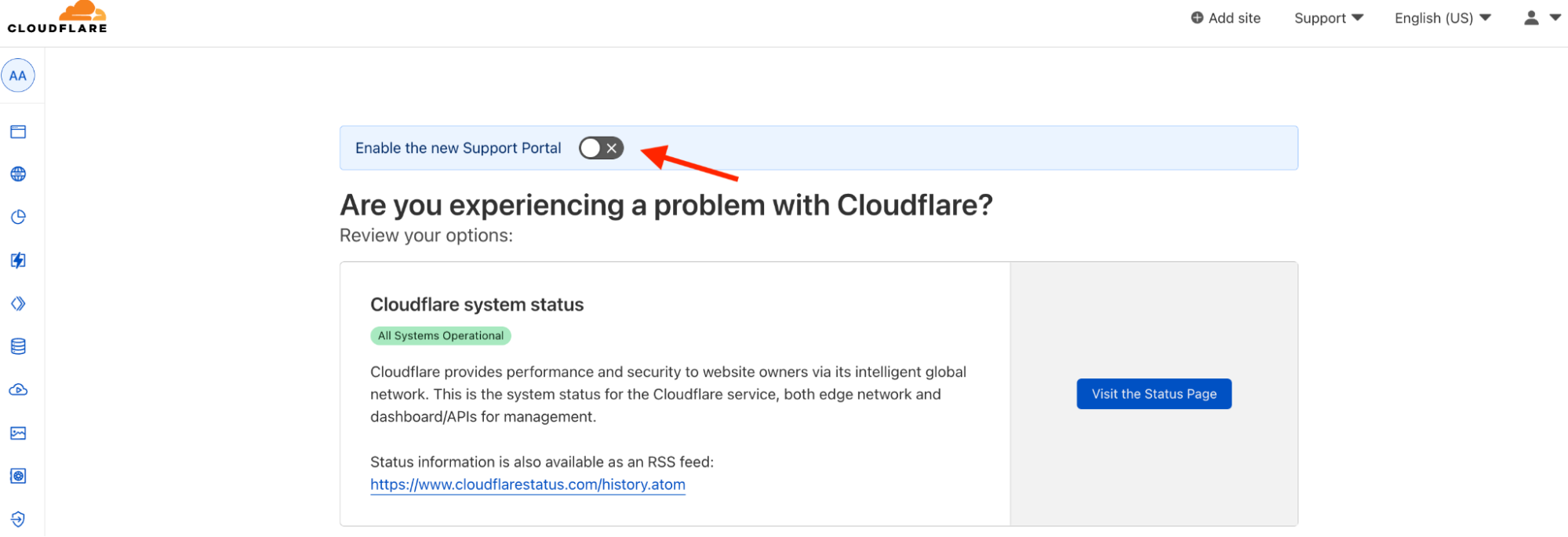The image depicts a CloudFlare website interface. At the top left corner, the CloudFlare logo is prominently displayed, featuring an orange and yellow illustrated cloud. To the right of the logo, there are several clickable buttons labeled "Add Site," "Support," "English," "US" (in parentheses), and a user icon depicting head and shoulders. Next to each button and icon, there are additional small rectangular or triangular icons.

On the left side of the screen, a vertical sidebar shows an array of blue icons, suggesting navigation options. The first icon is a circle with "AA" in it, possibly for accessibility features. The third icon down resembles a clock, likely representing a time-related function, and the fourth icon depicts a lightning bolt, possibly indicating speed or performance-related features.

Dominating the upper portion of the central display area, a rectangular blue bar reads, "Enable the new support portal," accompanied by a toggle switch that is currently in the off position. A large red arrow points towards this toggle switch, adding emphasis. Below this section, text inquires, "Are you experiencing a problem with CloudFlare?" and advises users to "Review your options." It further provides information about the CloudFlare system status, noting that "All systems operational." On the right side of this area, there's a blue box with the text, "Visit the status page," inviting users to check the detailed status.